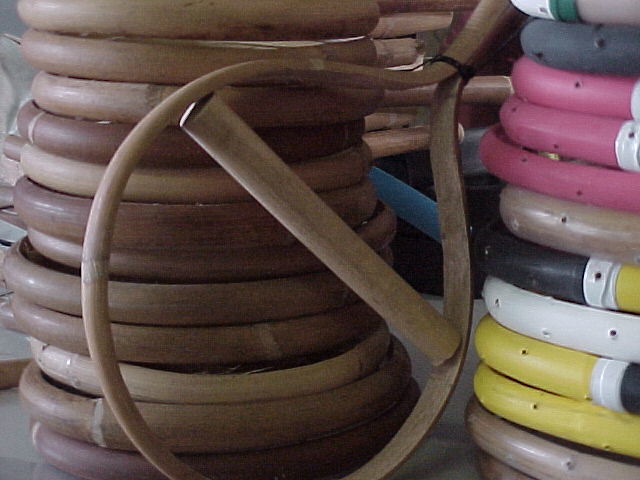The image depicts a close-up view of several round, wooden objects stacked in two distinct piles. These items resemble the base of a tennis racket, though slightly rounder and wider. Notably, a single wooden piece stands upright between the two piles for better visibility of its design, featuring a central cylindrical sidebar. The left pile consists of about a dozen natural-colored wooden items, while the right pile, partly cut off in the image, includes similar items that are painted in various colors such as yellow, pink, greenish-blue, white, and black. The scene appears well-lit, possibly taken under natural sunlight or with a flash, and the background is undisturbed, allowing full focus on the wooden objects. Their exact purpose remains unclear, adding an element of intrigue to the photograph.